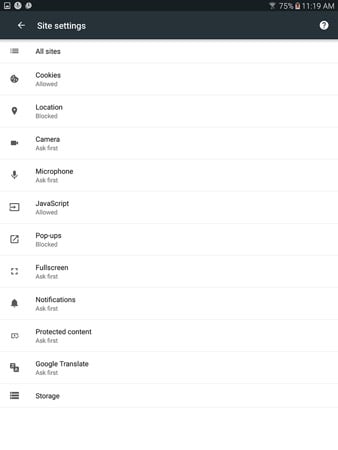A detailed screenshot from a smartphone displaying the "Site Settings" menu in the browser settings. At the top, a black bar shows it is 11:19 AM with 75% battery remaining and connected to Wi-Fi. The black bar also includes a header titled "Site Settings" alongside a back arrow for navigation. Directly below, a comprehensive list of various settings is visible, each separated by a faint gray line and accompanied by relevant icons. The list entries include "All sites," "Cookies" marked as allowed, "Location" marked as blocked, "Camera" set to ask before use, "Microphone" also set to ask first, "JavaScript" allowed, "Pop-ups" blocked, "Full screen" set to ask first, "Notifications" set to ask first, "Protected content" set to ask first, "Google Translate" set to ask first, and finally, "Storage." Icons next to each setting represent their respective functions, such as a bell for notifications, a location pin for location settings, a microphone icon for microphone settings, and a camera icon for camera settings.